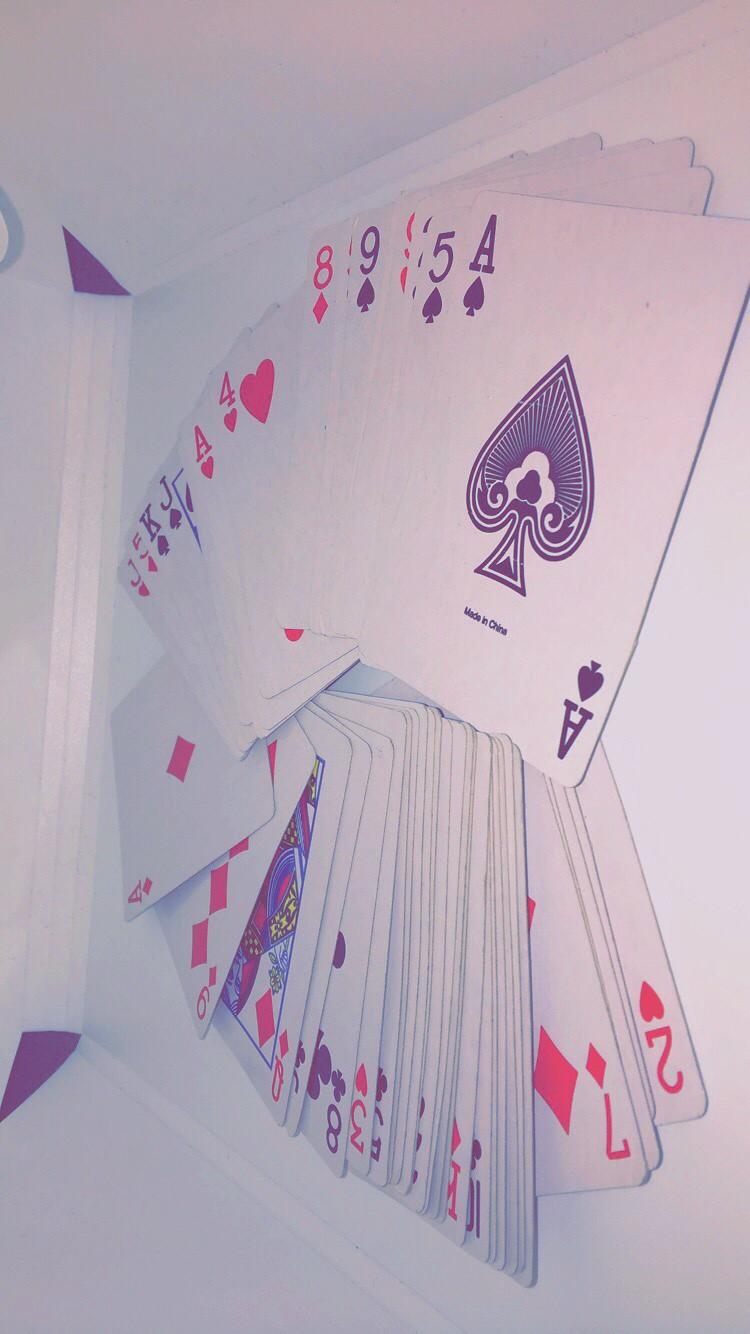In this photograph, a stack of playing cards has been meticulously fanned out in a semi-circular arrangement with their faces up, displaying a variety of cards in no particular order. Despite some cards being misaligned and bunched together, the deck reveals a mix of red and black cards prominently. Notable visible cards from top to bottom include: the black Ace of Spades, the Five of Spades, the Nine of Spades, the Eight of Diamonds, the Four of Hearts, the Ace of Hearts, the Jack of Spades, the King of Spades, the Five of Diamonds, the Jack of Hearts, the Ace of Diamonds, the Nine of Diamonds, the Queen of Diamonds, the Eight of Clubs, the Three of Hearts, the Seven of Diamonds, and the Two of Hearts. Among these mentioned cards, additional cards are partially visible but obscured, making their specific identities unrecognizable. The arrangement, containing approximately 50 to 52 cards, suggests it is a standard deck sans jokers. The pristine, durable condition of the cards—with no tears, marks, or visible fingerprints—indicates this is a well-maintained, possibly new deck of playing cards, fanned out elegantly to showcase their detail.